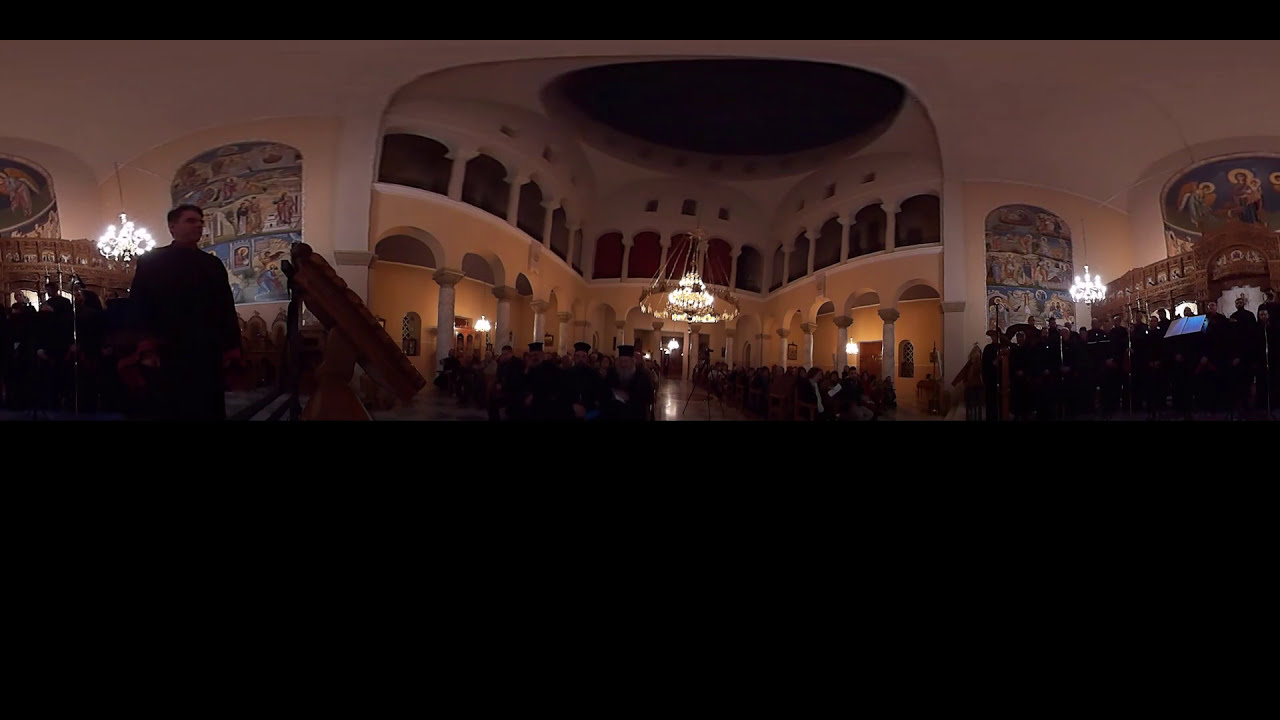The photograph captures the interior of an ornate building that resembles an opera house or a grand church. The spacious room is adorned with high cream-colored walls and supported by elegant pillars. Dominating the ceiling are chandeliers, intricately crafted with gold, casting bright light throughout the space. The image features two tiers: the ground floor, bustling with people, and an upper balcony lined with smaller arched pillars and red curtains, some of which are drawn open. The lower floor has open arches leading to further sections of the building. The scene includes several people seated and standing, lending to the bustling yet sophisticated atmosphere. Additionally, the room has a polished hardwood floor that glistens under the chandelier light. Seen from a panoramic perspective, the midsection of the ceiling features a circular design, and there are paintings on the walls, enriching the already lavish decor.